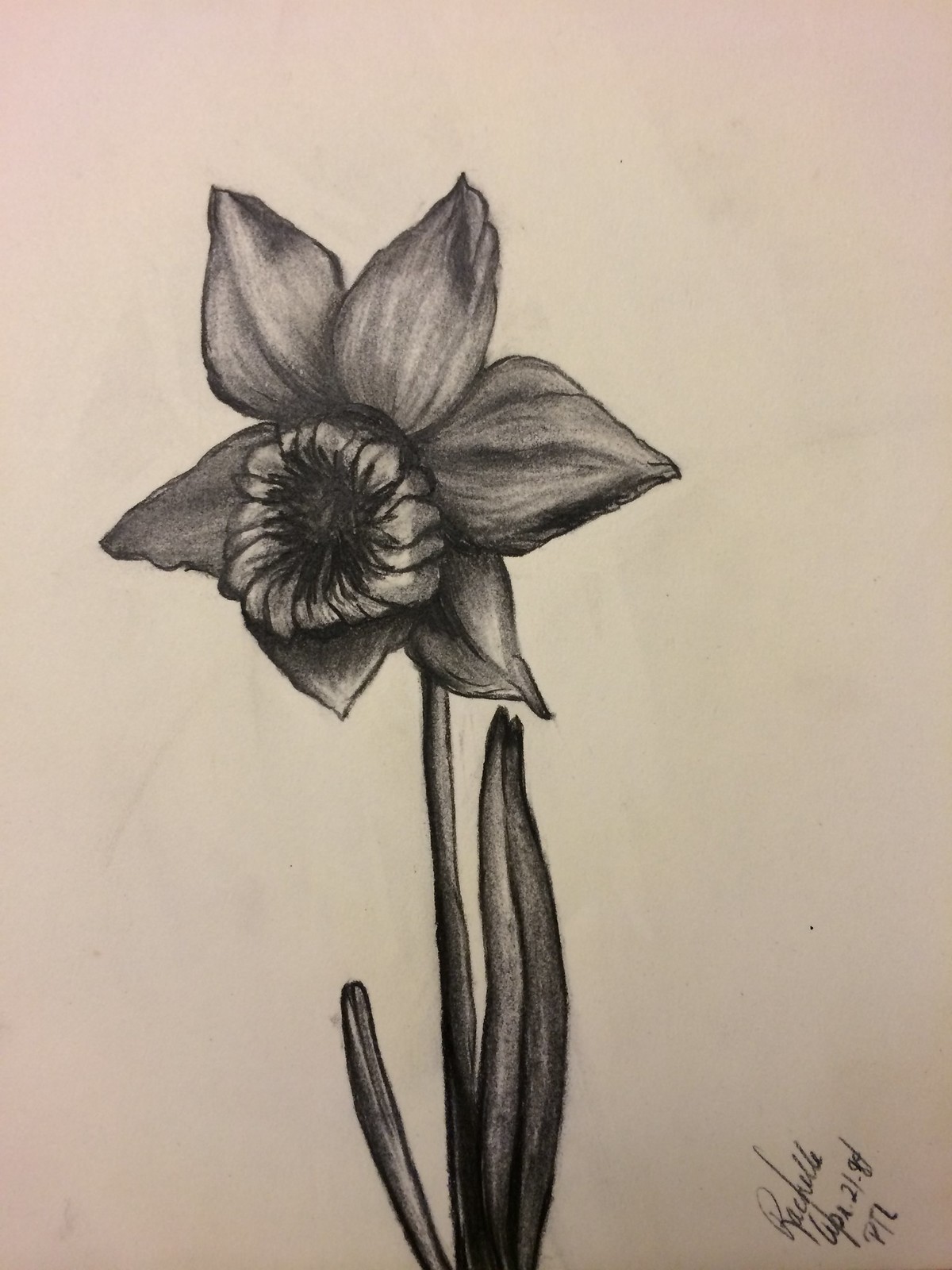The image is a hand-drawn, black-and-white illustration of a solitary flower, likely done in pencil. It appears to have been either photographed or scanned into a computer, and it sits on a beige background that has varying pinkish tones in the top left and bottom corners. The background is mostly beige, creating a subtle contrast with the black and gray hues of the drawing. 

The flower's stem is slightly undulated and supports two leaves. The taller leaf on the right nearly reaches one of the flower's petals at the top, while a smaller, thinner leaf on the left angles upward. The flower itself features six petals of unequal size, surrounding a pronounced central head where the pollen would be, characterized by detailed shading.

In the bottom right corner is a stylized signature, written in cursive at an angle requiring a 45-degree tilt to the left to read clearly. The signature appears to read "Rochelle Lippa," with "Rochelle" on the top line and "Lippa" on the second line, followed by what looks like the date "2-1-89" or possibly a similar variation if the last two digits are not clear. Underneath this date, the letters "P-I-Z" (or perhaps "P-T-L" based on interpretation) are inscribed.

Overall, the detailed shading and realistic portrayal give the flower a vibrant and healthy appearance, despite the monochromatic color scheme.